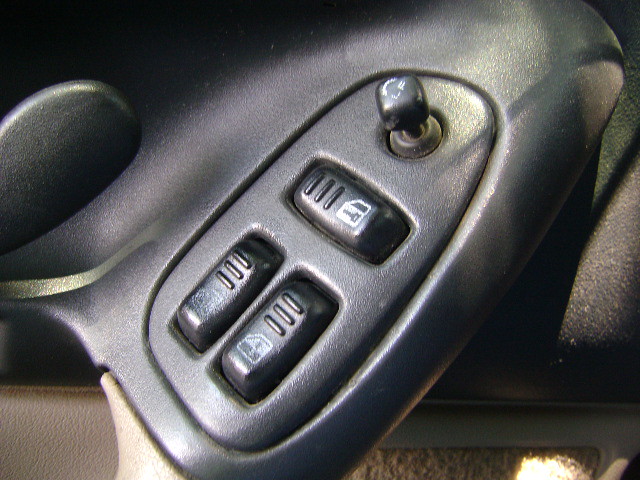The image captures a detailed view of the interior of an older car's door, focusing specifically on the control panel. The panel features a mix of black, thick plastic materials, and you can see a carpety-looking tan material at the bottom right, likely part of the floor or side panel. The controls include several buttons and switches: a black toggle at the top, likely for adjusting the side mirrors; a black button with an icon resembling a key and lock, used for locking and unlocking the doors; and two additional black switches characterized by raised ridges, presumably for rolling the windows up and down. The design and layout of these controls suggest a vintage car model.